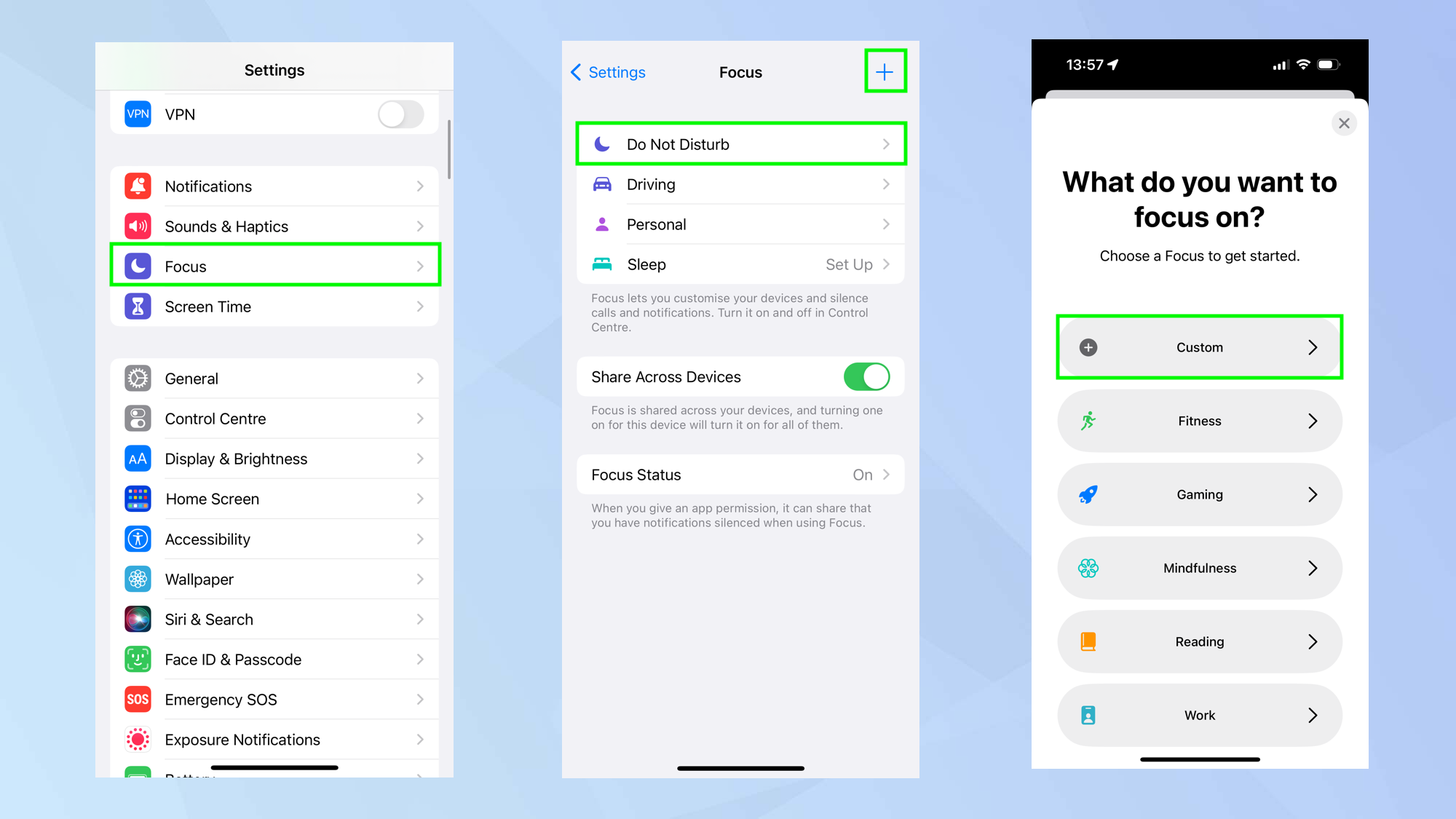This is a photograph displaying three sequential screenshots set against a light blue background embellished with a faint geometric pattern. 

1. The first screenshot captures the "Settings" menu on a mobile device. The "Focus" section is highlighted with a neon green overlay, indicating it is selected. Other visible menu options include "Notifications," "Sounds & Haptics," and "Screen Time," accompanied by general controls and the home screen settings listed below.

2. In the second screenshot, the "Focus" section is fully opened. At the top left, a blue arrow pointing left signifies the option to navigate back to the previous settings menu. In the upper right corner, a plus icon, also highlighted in neon green, marks the area to add a new focus mode. Below are various focus modes listed, such as "Do Not Disturb" (with a moon icon), "Driving," "Personal," "Sleep," and others. The "Do Not Disturb" mode is selected, as indicated by the neon green highlight surrounding it.

3. The third screenshot features a pop-up titled "Choose Your Focus" with an 'X' icon in the upper right corner for closing the dialog. The pop-up prompts the user to select a focus mode to get started, presenting options like "Custom," "Fitness," "Gaming," "Mindfulness," "Reading," and "Work." The "Custom" option is selected, as denoted by the same neon green rectangular highlight. 

This detailed depiction conveys a clear visual narrative of navigating through and selecting various focus modes on a mobile device.